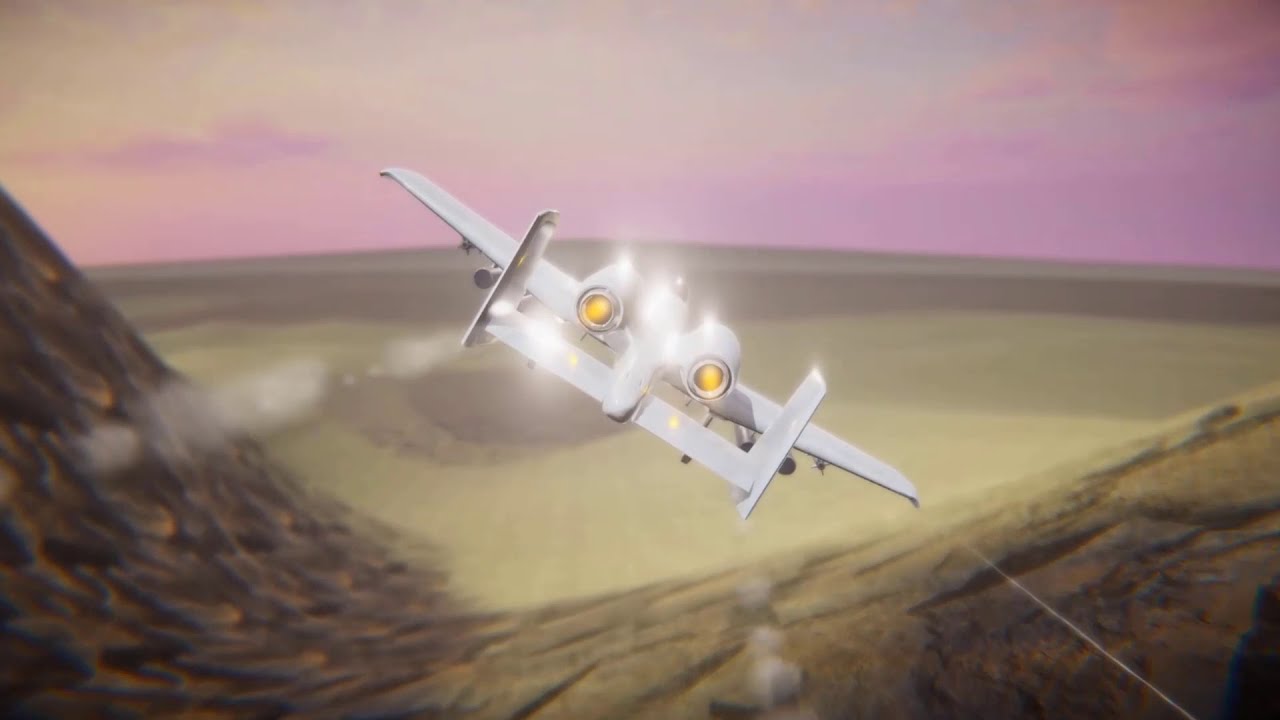The image is a detailed 3D rendering, possibly from a video game or an animated cartoon, showcasing a military aircraft flying over a vast, deserted, mountainous area. The aircraft, likely a fighter jet, is seen from the back and is light gray or white in color with highly reflective surfaces. It is centered in the image, angled as if making a right turn, with the left wing pointing up toward the top left and the right wing angled down towards the bottom right. The jet has twin engines at the rear, emitting bright, yellow-gold flames or homage flames, and possibly some smoke or sun reflections. It features a narrow body, two vertical fins, a horizontal stabilizer at the back, and visible missiles and armaments under its wings. The sky overhead is a striking mix of pink, purple, and white hues, adding to the dramatic effect. In the foreground, the jet flies over steep hills and through a canyon or valley, with the distant background revealing a flat, barren landscape of deserts and dunes. The juxtaposition of colors in the scene includes shades of pink, white, silver, tan, brown, black, and yellow.